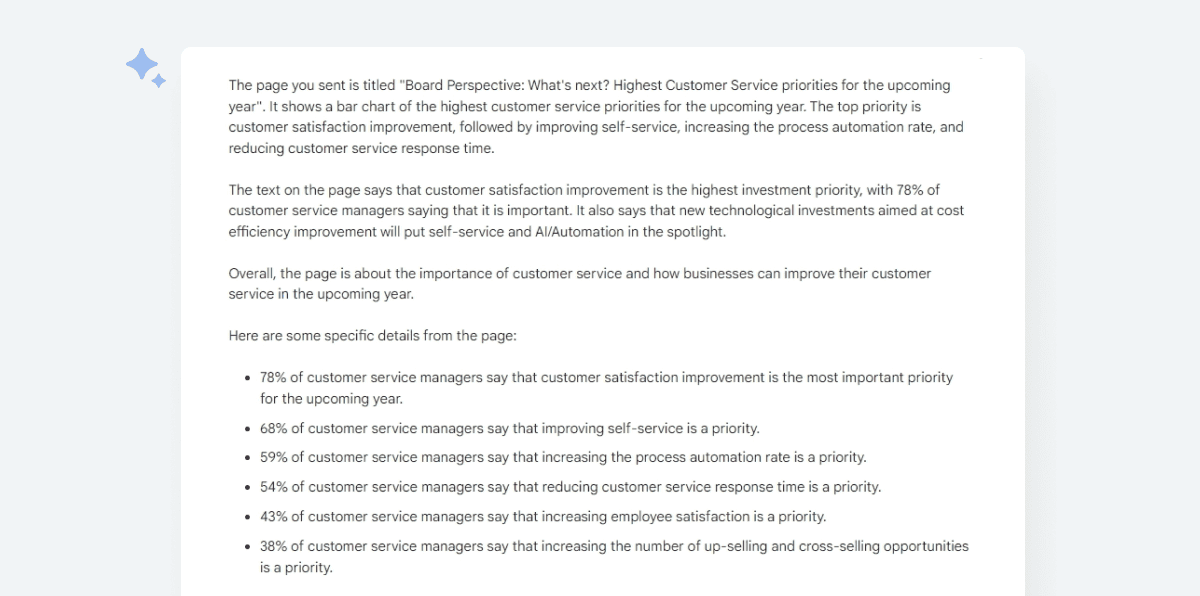### Descriptive Caption:

This image is a detailed screenshot of a document, presumably generated by AI, as indicated by the two stars in the upper left-hand corner. The document is displayed on an off-white, eggshell-colored background, with the text in a small, approximately size-8 font. The document is titled "Board Perspective: What's Next? Highest Customer Service Priorities for the Upcoming Year."

In the upper portion, the document features a bar chart illustrating the highest customer service priorities for the upcoming year. The chart highlights the following key priorities:
1. Customer satisfaction improvement.
2. Improving self-service.
3. Increasing the process automation rate.
4. Reducing customer service response time.

Below the bar chart, a detailed explanation states that customer satisfaction improvement is the highest investment priority, with an impressive 78% of customer service managers identifying it as crucial. It further explains that new technological investments aimed at enhancing cost efficiency will shine a spotlight on self-service and AI/automation.

The document elaborates on the importance of customer service and how businesses can enhance it in the upcoming year. Key details mentioned include:

- **68%** of customer service managers prioritize customer satisfaction improvement.
- **68%** also emphasize the importance of improving self-service.
- **59%** prioritize increasing the process automation rate.
- **54%** focus on reducing customer service response time.
- **43%** consider increasing employee satisfaction important.
- **38%** believe increasing the number of upselling and cross-selling opportunities is crucial.

Overall, the page underscores the strategic areas where businesses plan to invest in order to elevate their customer service performance in the year ahead.